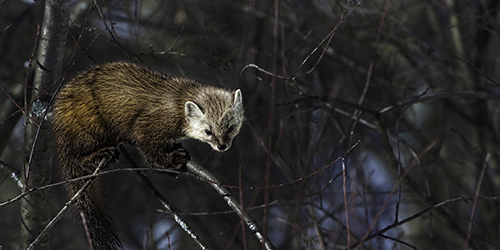In this outdoor image, amidst a backdrop of blurred, grayish-brown bare tree branches that form a maze-like pattern, a thick-furred animal clings to a thin tree branch. The background hints at the possibility of snow-covered ground or light-colored soil, adding a cold and wintry atmosphere. The creature has a distinct appearance with an upside-down triangular head that is round and short, adorned with whitish fur on its face, black eyes, small ears that appear almost like eyebrows, and a short snout. Its body is covered in dense, brown fur tipped with black hair, making it look incredibly thick and well-insulated. The animal possesses short legs and a long, black tail that hangs down from the branch, which adds to its unique and striking appearance.